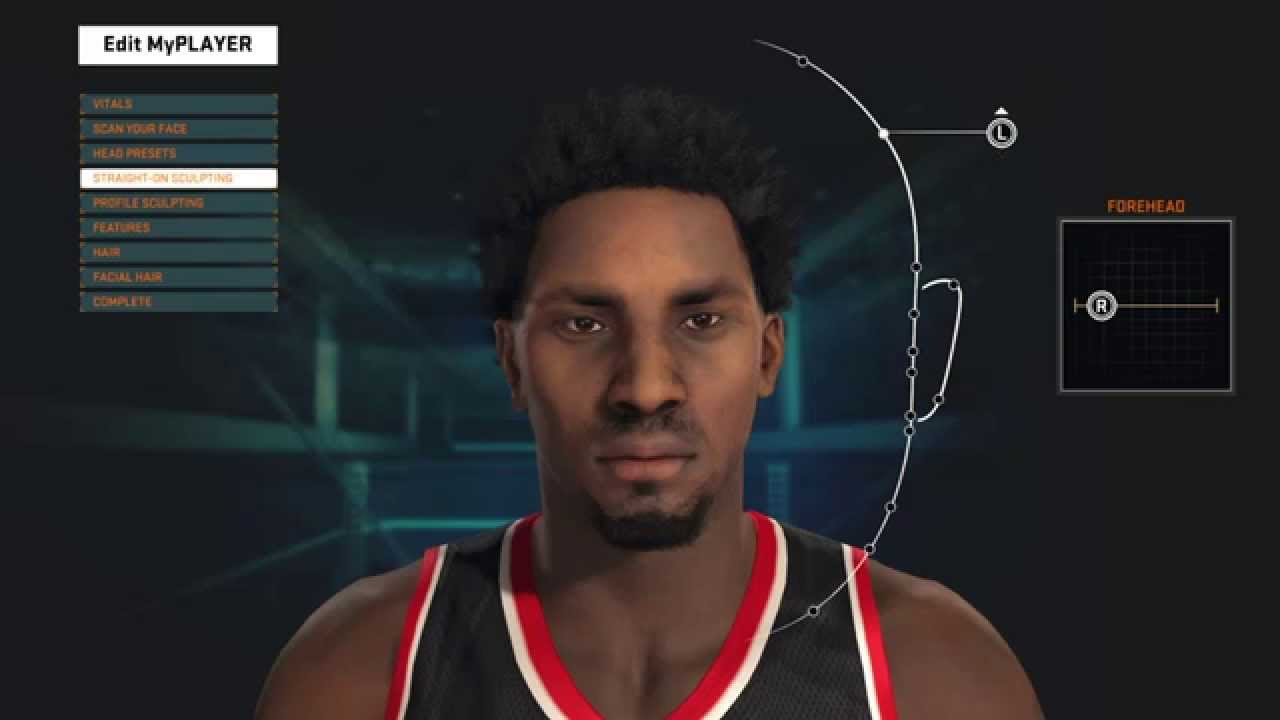The close-up image features a basketball player, showcasing his face, shoulders, and the upper part of his chest. He is donned in a black basketball jersey with red trimming along the outer edges, and white lining the inner parts of the edges. The player has black hair and sports a distinct goatee, which is slightly longer around his chin.

The image has a stylized element to it, with a white line silhouette tracing the right side of his face, giving it an almost hand-drawn appearance. Intriguingly, there is a round button near the silhouette with an 'L' in the center, connected by an upward-pointing arrow to the line outlining his face. Additionally, a vertical menu labeled "Edit My Player" is present in the upper left-hand corner of the image.